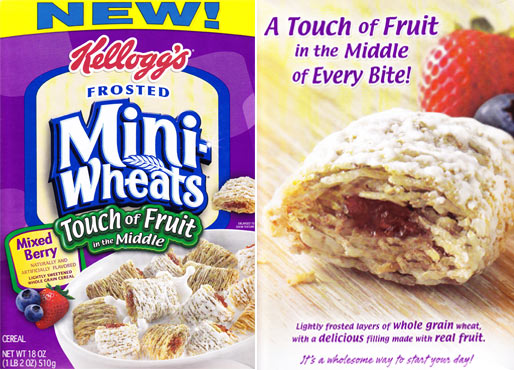The compilation features two detailed images of the Kellogg's Frosted Mini-Wheats cereal box. 

**Left Image:**
The left image showcases the front of the cereal box, prominently featuring Kellogg's Frosted Mini-Wheats with the flavor described as "A Touch of Fruit in the Middle: Mixed Berry." The box illustration clearly emphasizes the innovative twist on the classic Mini-Wheats, highlighting that each cereal piece has a mixed berry fruit filling, comprising strawberries and blueberries. This front panel has the usual branding and graphics found on cereal boxes, making it easily recognizable.

**Right Image:**
The right image appears to be the side label or back of the box, providing further description and visual details. Centrally displayed is a single Mini-Wheat cereal piece, split open to reveal the fruity filling inside. Surrounding this visual, to the top right, are enlarged images of a strawberry and a blueberry, underlining the mixed berry flavor. At the top of this image, the text reads, "A touch of fruit in the middle of every bite," followed by a description below that states, "Lightly frosted layers of whole grain wheat with a delicious filling made with real fruit. It's a wholesome way to start your day." This descriptive breakdown projects the cereal's wholesome and flavorful appeal.